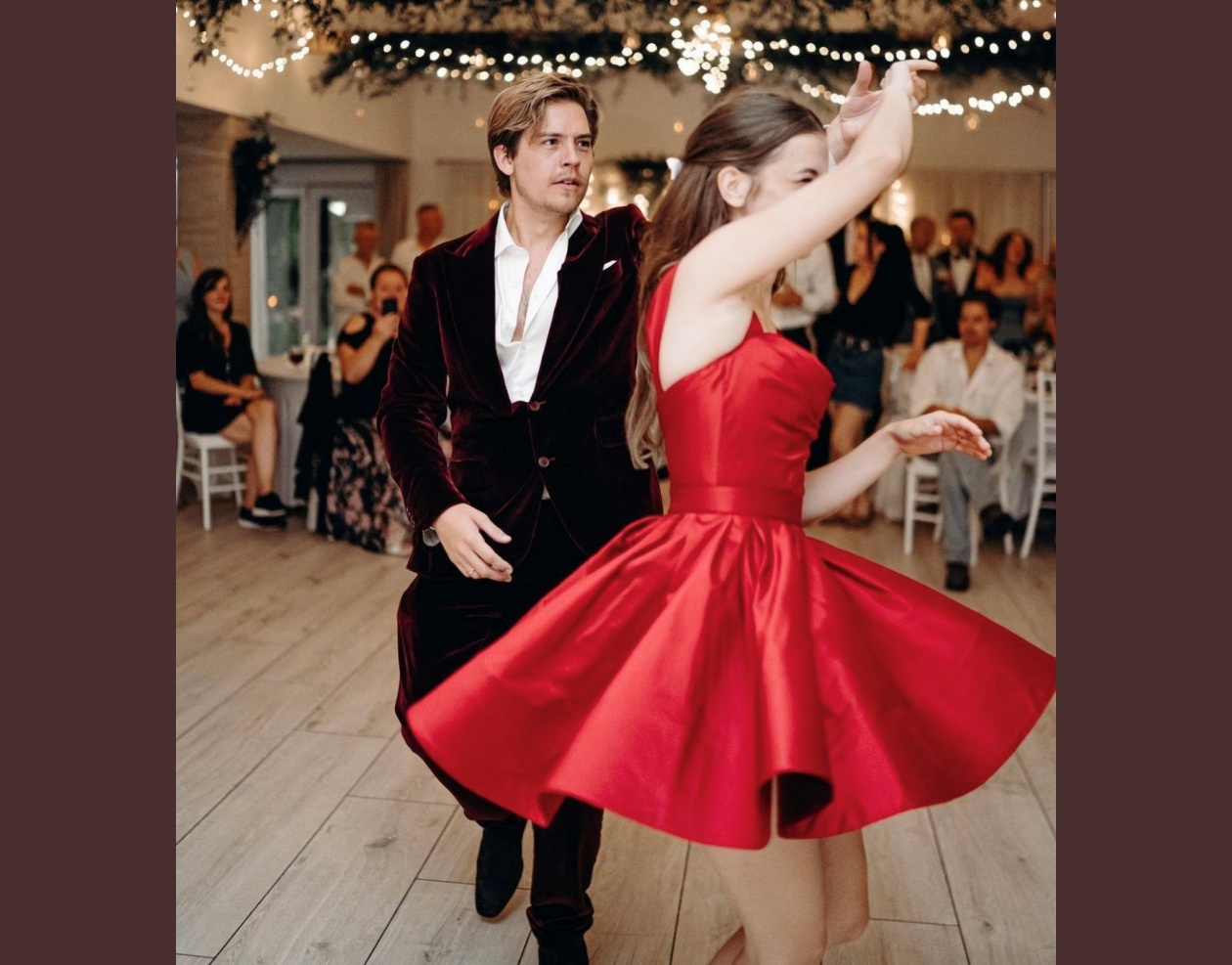In this vibrant and festive indoor setting, a young couple, possibly in their late 20s, are the center of attention as they dance gracefully on a light brown hardwood floor. The man, on the left, is dressed in a black tuxedo with a white unbuttoned shirt and longish dyed blonde hair. Notably, he is missing a tie. Beside him, the woman twirls in a bright red satin dress with a short and flared skirt, her long brown hair pulled back elegantly. She raises her right arm above her head while her left arm stays bent by her waist, holding the man's hand. Behind them, several people are seated at white tables and chairs, watching the dancers with intrigue. Overhead, garlands adorned with twinkling white lights add to the festive atmosphere. The image is bordered by purplish-brown vertical stripes, enhancing its rectangular frame, and is a perfect representation of a joyous celebration captured in a moment of time.